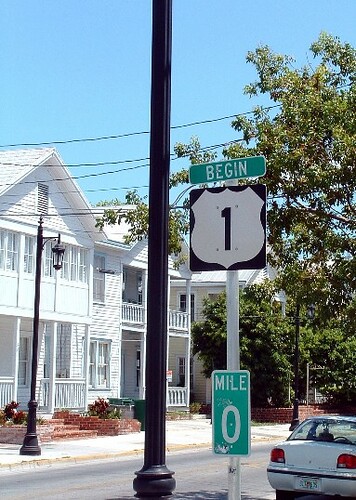This rectangular, portrait-view photograph captures a charming street scene with several distinct elements. In the foreground, a street sign prominently displays the word "BEGIN" atop a pole, followed by a white number "1" on a black background, and "MILE 0" in white text over a green background. Black streetlights line the road, adding an element of symmetry and structure to the scene. To the left, a large white house with classic architectural features stands out against the backdrop of medium green trees. In the bottom right corner, a white car is partially visible, adding a touch of modernity. The light blue sky overhead brings a sense of tranquility and openness to this picturesque streetscape.